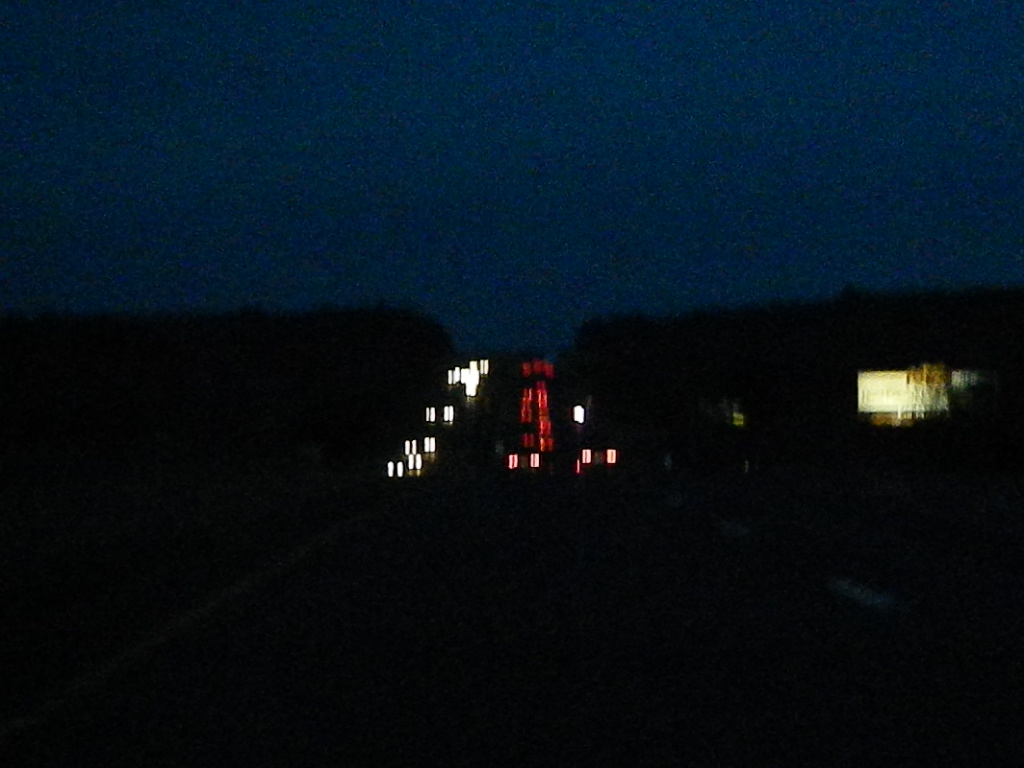A nighttime photograph captures the dynamic flow of traffic ascending and descending a hill. Positioned parallel to the road, the photographer encapsulates a stream of oncoming headlights and departing taillights, each reduced to distinct pairs of white and red dots, respectively. Despite the extreme blur, the image distinctly portrays a busy roadway. The land beneath is shrouded in pitch-black darkness, contrasting sharply with the navy blue expanse of the sky above. To the right of the scene, a blurred rectangle of light suggests the presence of a billboard, adding an element of urban life to this nocturnal traffic scene.